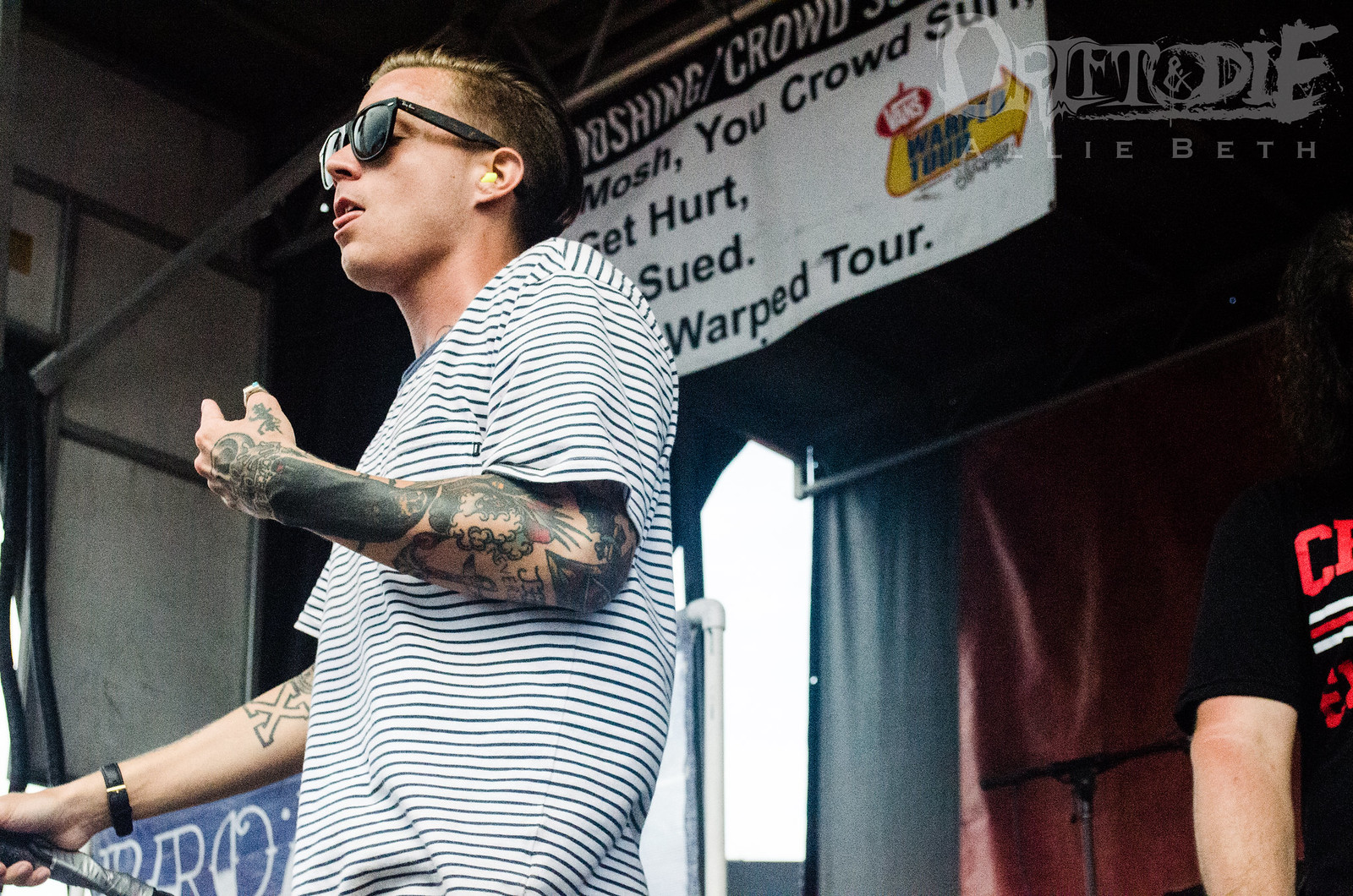The photograph captures a vibrant, detailed scene at an outdoor music concert, likely the Warped Tour. Center stage stands a young, heavily tattooed music artist, dressed in a white t-shirt with black horizontal stripes and black Ray-Ban Wayfarer sunglasses. His short light brown hair and Caucasian features are distinctly visible. With his right hand, he grips a microphone stand, noticeably wrapped in duct tape, while his left hand, adorned with extensive tattoos, gestures animatedly towards himself. The artist's intent gaze is directed at the crowd.

The backdrop reveals a makeshift stage construction: a wooden side wall with metal framing on the left, a large black tarp covering a red one at the rear, and a visible gap above that shows the blue sky, confirming the outdoor venue. Suspended above the stage is a partially visible banner that cautions the audience with the words, "you mosh, you crowd surf, get hurt, get sued," and references to the Warped Tour. Slightly to the right of the main performer, another individual can be seen partially; he wears a black t-shirt with only his right arm in view. In the top right corner of the photo, the text "Drift and Die, Alley Beth" is faintly visible, adding an intriguing detail to the energetic, bustling atmosphere of the concert.